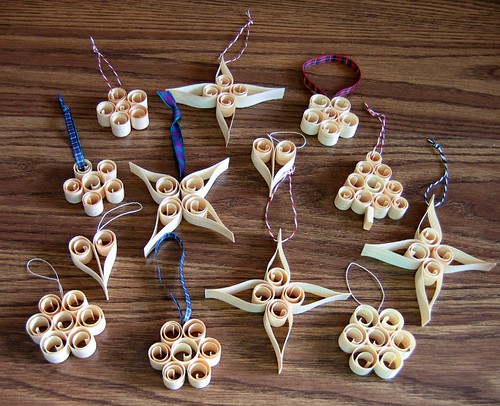The photograph showcases an assortment of delicate, handmade ornaments positioned on a medium walnut brown wooden table with horizontal grain patterns. These ornaments, crafted from rolled paper resembling cylindrical shell shapes, bear a festive resemblance to Christmas decorations. Each ornament is affixed with a variety of ribbons and strings, including blue, red and white, blue and white, plain white, and a purplish string for hanging.

Among the ornaments, several distinct shapes are identified: there are two heart-shaped ones, up to six configured like flowers, and at least four fashioned into star-like or snowflake designs. Notably, a Christmas tree-shaped ornament with an additional small piece of wood representing the trunk stands out, adorned with a purple and white string.

In the top row of the image, three ornaments are displayed, including a flower-shaped and a butterfly-like design with four projections. The second row mirrors these patterns with an additional ornament resembling two eyes with an inverted triangle, alongside a Christmas tree. The lower sections of the image continue with variations of the flower and butterfly designs, completing a visually appealing arrangement of approximately ten intricate ornaments.